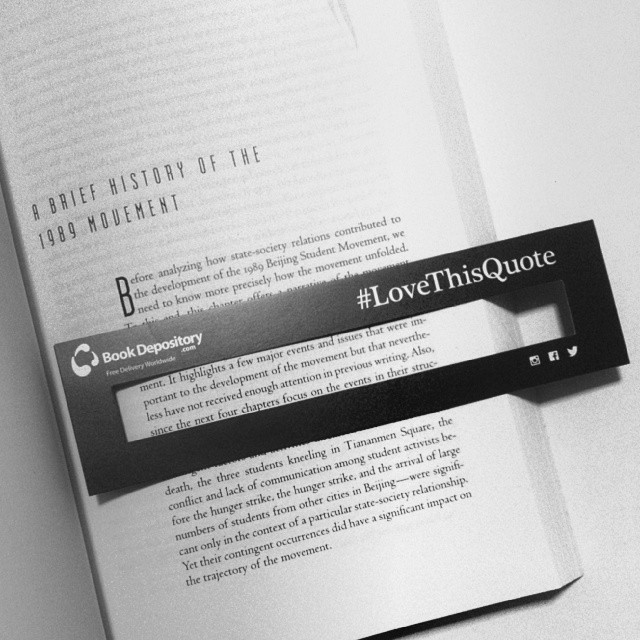This black-and-white photo features an open book lying on a whitish-gray table. The book is turned to the start of a chapter titled "A Brief History of the 1989 Movement." On the open page, there is a black bookmark overlaying the text, drawing focus to a specific quote. The highlighted quote reads: "It highlights a few major events and issues that were important to the development of the movement, but that nevertheless have not received enough attention in previous writing. Also, since the next four chapters focus on the events in their structure..." The bookmark itself has a rectangular opening to aid in reading the highlighted text. On the top left of the bookmark, it reads "bookdepository.com." To the right, in larger white font, the bookmark bears the hashtag "#lovethisquote." At the bottom of the bookmark are social media logos, including those for Instagram, Facebook, and ex-Twitter, marking the intersection of literature and social media engagement in this visually striking image.